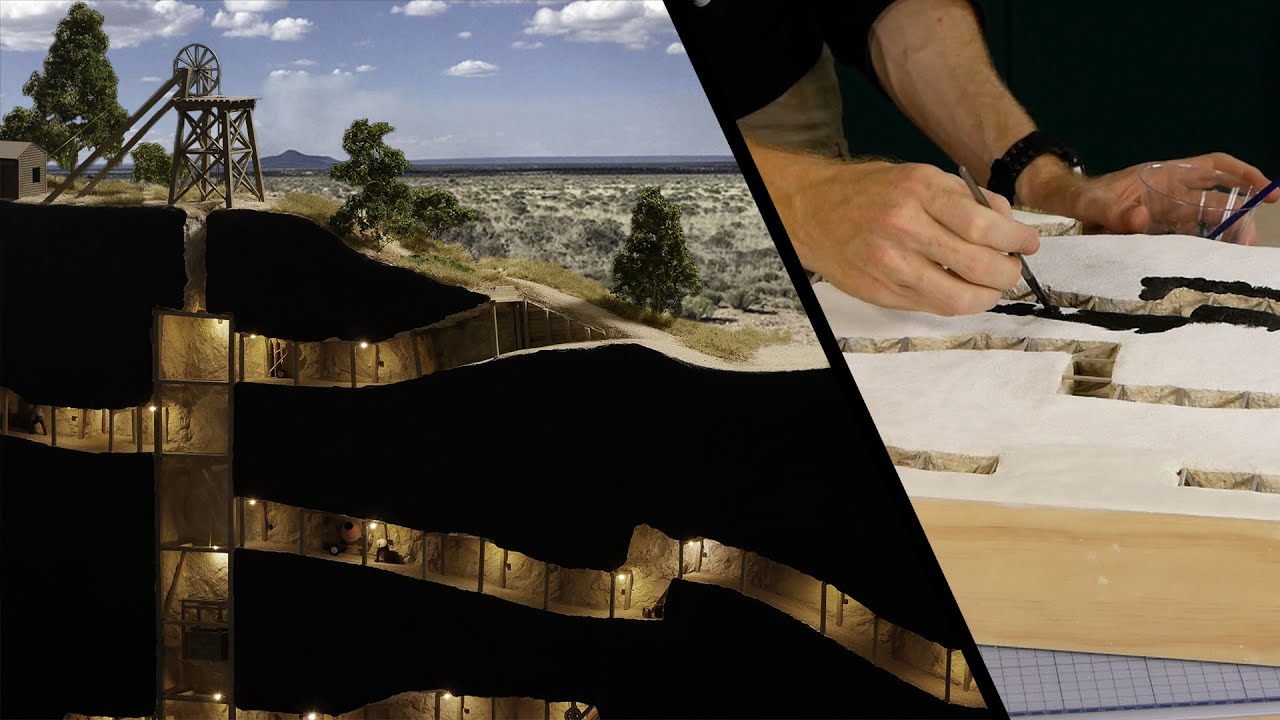The image is a two-part collage. On the left, it vividly depicts a realistic scale model of a desert landscape with a well atop a hill under a sunny sky with clouds. Below the well, the model reveals various layers of a mine, complete with illuminated tunnels that give off a golden hue, contrasting with the black surroundings that emphasize the underground aspect. The scene captures an intricate blend of surface realism and subterranean complexity. On the right, the creation process is documented, showing a man's hands—wearing a black watch on his left wrist and a black t-shirt—meticulously painting the white surface of the model. He uses black paint to define the channels and tunnels within the mine, bringing the underground landscape to life. The right image provides a behind-the-scenes glimpse into the careful artistry involved in crafting the detailed topography depicted on the left.